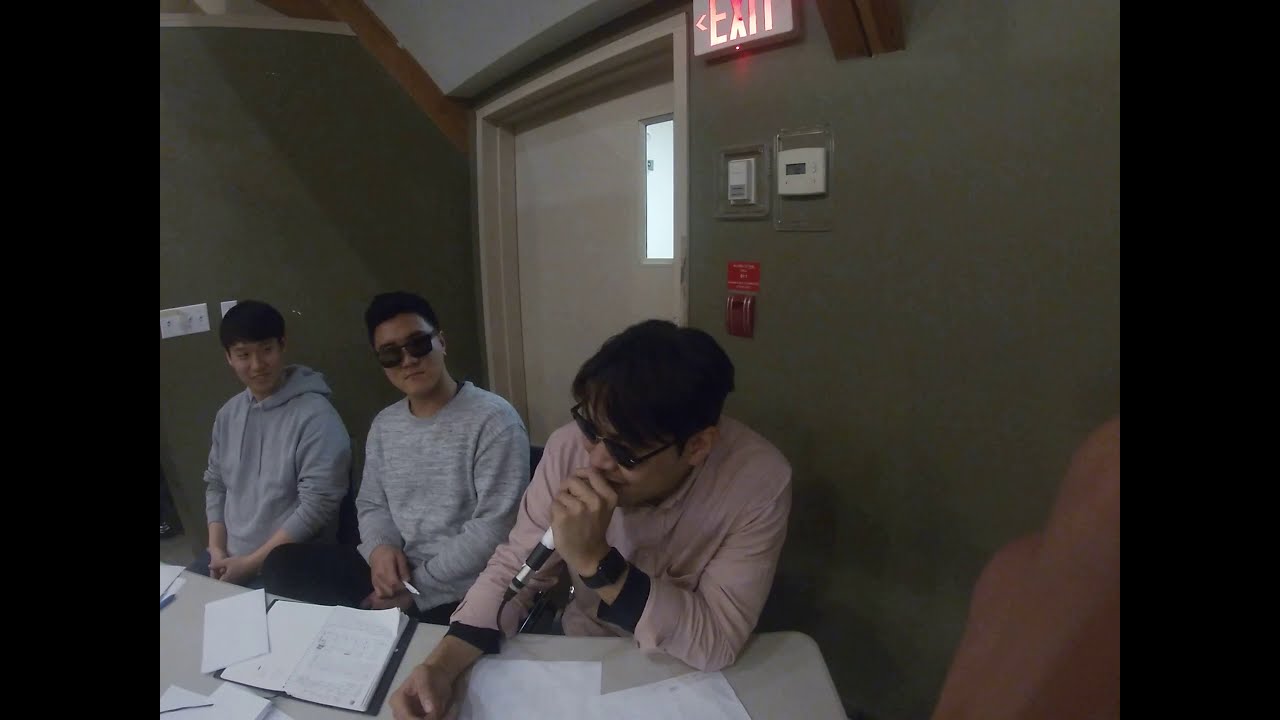The photograph is a rectangular indoor shot capturing a room with army green walls and a white door in the background, topped by an exit sign. Standard wall fixtures such as a thermostat and fire alarm are also visible. Seated at a desk laden with an assortment of papers, notebooks, and envelopes are three Asian men. The man on the far left is wearing a gray hoodie and is looking towards the center, where another man is seated in a gray sweatshirt and dark sunglasses, casually leaning his elbow on the desk. The third man, on the far right, is dressed in a pink button-down shirt and dark sunglasses, holding and speaking into a microphone. His body is angled slightly forward, engaging in what appears to be a discussion or possibly recording a podcast or radio show.